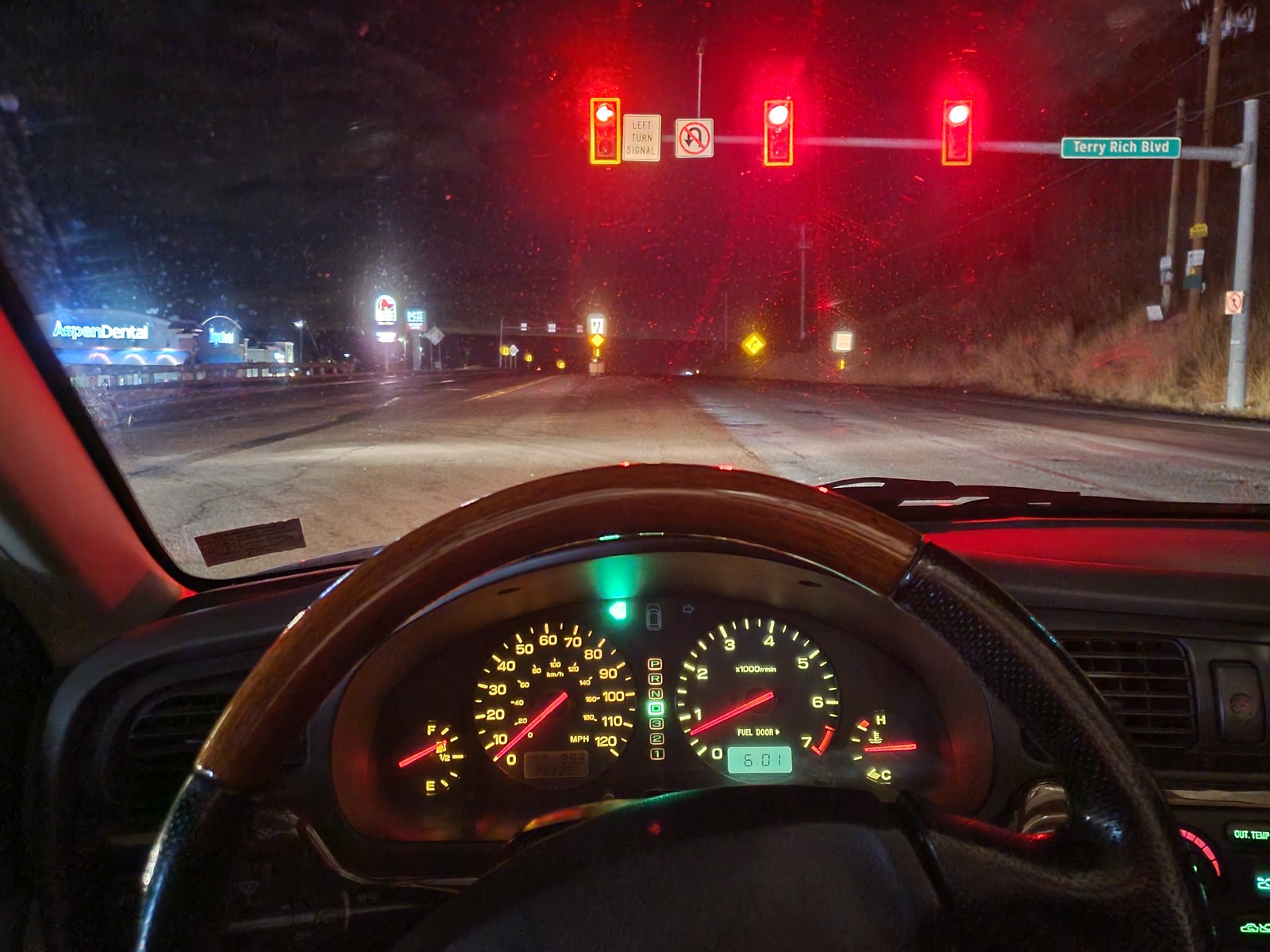This detailed photograph captures the inside of a car at night, viewed from the passenger seat. The instrument panel is illuminated with yellow numbers and letters, indicating the speedometer, fuel gauge, and coolant gauge (marked with "C" for cool and "H" for hot). The speedometer features smaller yellow numbers for kilometers per hour, and the fuel gauge has a red arrow, similar to the speedometer. The gear indicator shows squares for park, reverse, neutral, drive (illuminated in green), and the numbers 1, 2, and 3. A green turn signal arrow is displayed at the top, indicating a left turn. The dashboard, a combination of wood and black materials, reflects the red glow of the stoplight.

The car is stationary at a red light on Terry Rich Boulevard, as indicated by a green rectangular street sign with white text and border. Adjacent to the street are traffic signs, including one forbidding U-turns and another directing a left turn at the signal. Additionally, there is a distinct red "No U-turn" sign. In the distance, a retail area with an illuminated blue sign for Aspen Dental is visible, featuring gray frontage and dark blue arches. The background comprises a hillside with telephone poles, further emphasizing the vehicle's nocturnal setting.